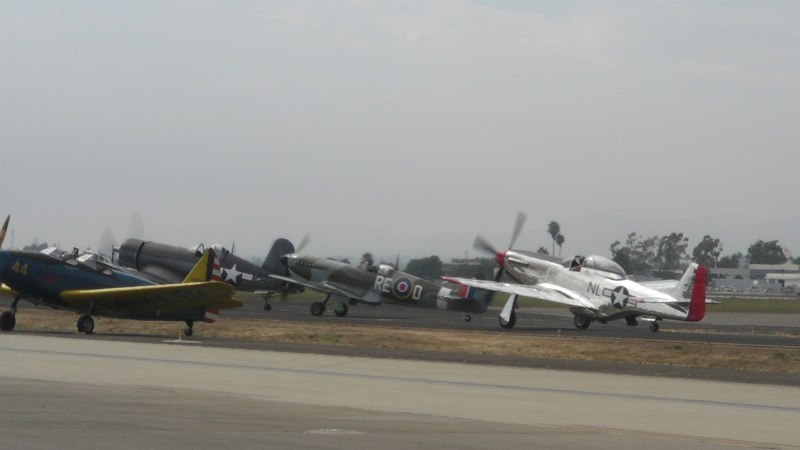This photograph, captured in an outdoor setting, showcases four vintage military aircraft with spinning propellers, suggesting they are either on the runway or preparing to take off. The planes, characterized by their distinct colors and markings, seem to be part of an air show performance. The aircraft appear well-maintained, harking back to several decades ago and exude the aura of classic fighter planes. The plane on the far left is adorned in blue and yellow, while the next one is a solid slate gray. The third plane features a gray and brown camouflage pattern, and the rightmost aircraft is primarily white with red trim and a distinctive blue circle with a white star. The airstrip is lined with a gray tarmac and a strip of browned grass, indicating a possible fall or early winter season. The backdrop includes a hazy, tropical sky with palm trees visible in the distance. The propellers blur with motion, indicating the planes are gearing up for their upcoming performance.